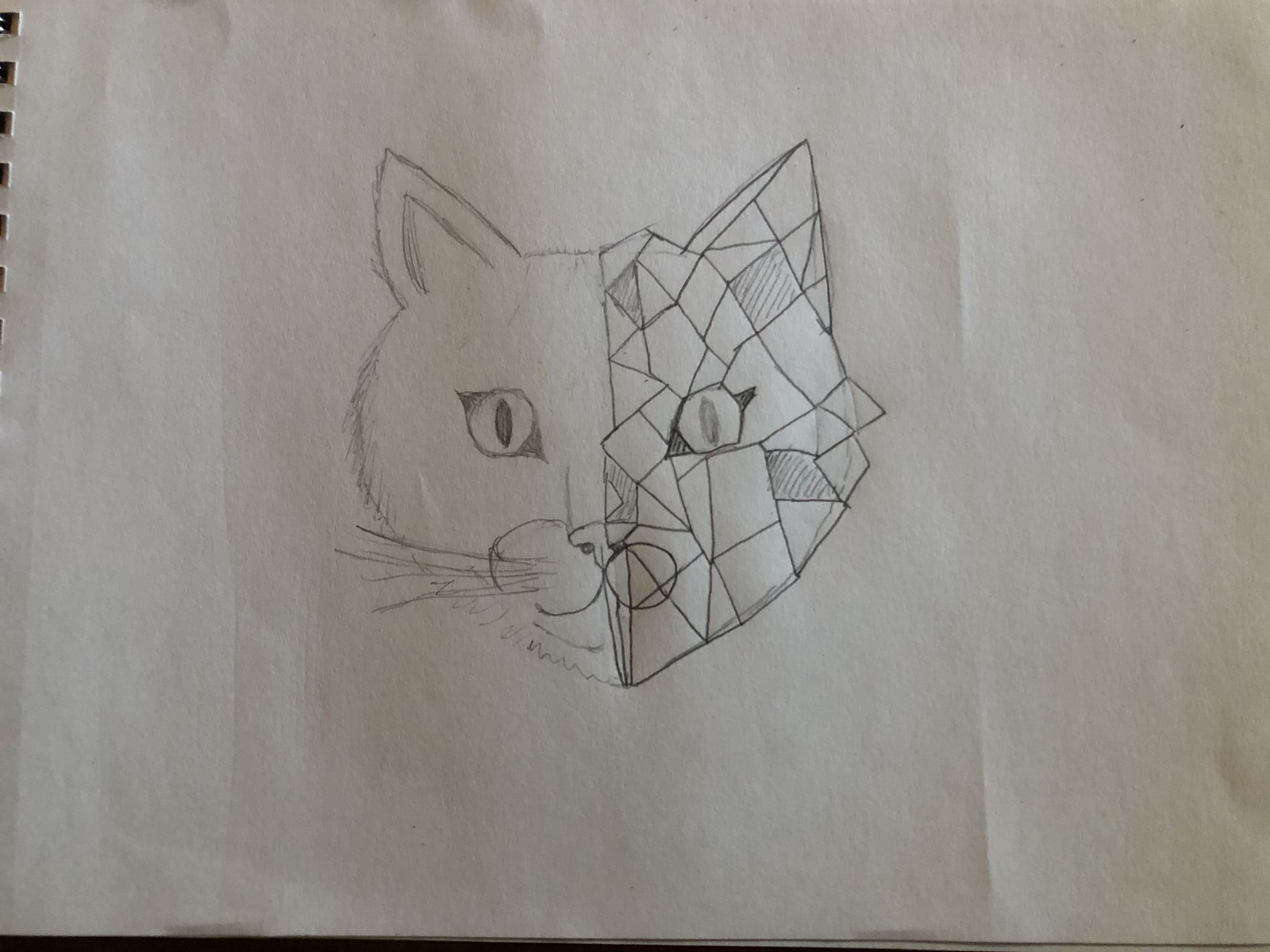The image features a detailed pencil and pen sketch of a large cat's head on a crinkled and shadowed white piece of paper. The background includes some faint visible rings of a binder in the upper left corner and a dark, shadowed area at the bottom. The left side of the cat's face is rendered in pencil, showing a naturalistic depiction with intricate shading, complete with a pointed ear, four whiskers, an eye with a sharp black pupil, and detailed fur. In contrast, the right side of the face appears crystallized or stained glass-like, created with black pen and filled entirely with geometric squares. This side lacks whiskers and fewer facial details, offering a stark artistic juxtaposition to the more realistic left side, encapsulating both traditional and abstract art styles in a single cat illustration.